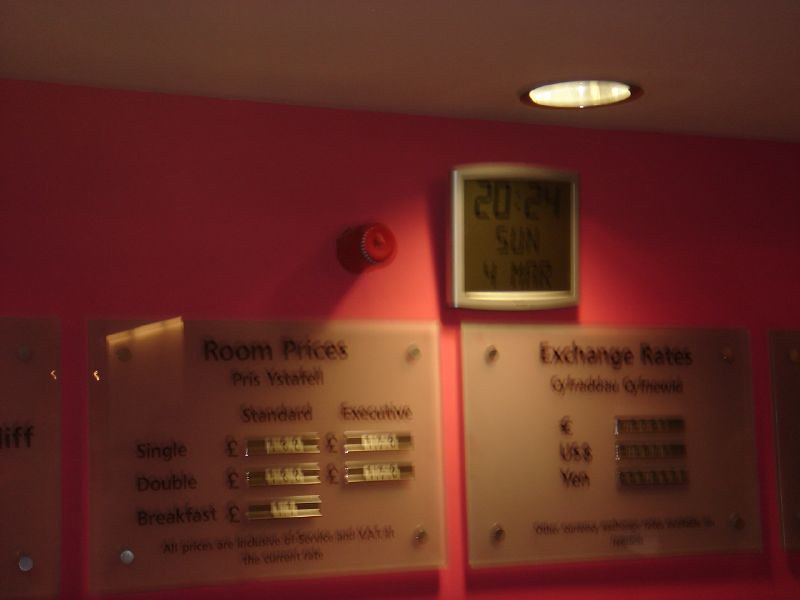This image captures the somewhat blurry interior of what appears to be a dimly lit room, possibly a hotel lobby. The ceiling, which is either brown or gray, has a spotlight in the center, casting light down into the room. On the red wall, a prominent digital clock displays "20:24" along with "Sunday" and "March 4th." To the left of the clock, there is what looks like a fire alarm or detector. Below the clock, several rectangular, transparent plastic signs with dark prints are clearly bolted to the wall. The sign on the left is for "Room Prices," listing categories such as "Standard" and "Executive" with options for "Single," "Double," and rooms that include breakfast. The adjacent sign on the right displays "Exchange Rates" for currencies like the Euro, U.S. Dollar, and Yen. Despite the photograph's lack of clarity, the basic information about room categories and exchange rates is discernible.